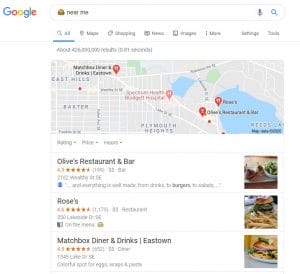In the Google search results page, the search query "French fries near me" is prominently displayed in black text within the search box. Right below this, the menu options are visible, including "Maps," "Shopping," "News," "Images," followed by a "More" option denoted by three vertical dots. Towards the right-hand corner, you see options for "Settings" and "Tools."

In the top left corner of the page, the iconic multi-colored Google logo is visible, with the uppercase 'G' in blue, the first 'o' in red, the second 'o' in yellow, the 'g' in blue, the 'l' in green, and the 'e' in red.

Dominating the page is a map with various streets delineated by white lines, light blue areas indicating bodies of water, and several red pins marking restaurant locations. Below the map, there are three gray dropdown menus labeled "Rating," "Price," and "Hours."

The first listing is "Olive's Restaurant and Bar," displayed in bold black text. To the right, there is a small image showing a side salad and two other dishes. Below this listing is another one labeled "Roses," accompanied by an image of a hamburger with French fries.

Further down, "Matchbox Diner and Drinks" is listed, separated from the previous entries by a line divider and also marked with "East Town." An image to the right of this listing depicts a hamburger with a pickle on top.

"Olive's Restaurant and Bar" boasts a 4.5-star rating, displayed with five star icons, four and a half of which are colored orange. The address and a brief description of the restaurant are provided in light gray text. Similarly, "Roses" has a notable 4.6-star rating, while "Matchbox Diner and Drinks" features the rating prominently as well.